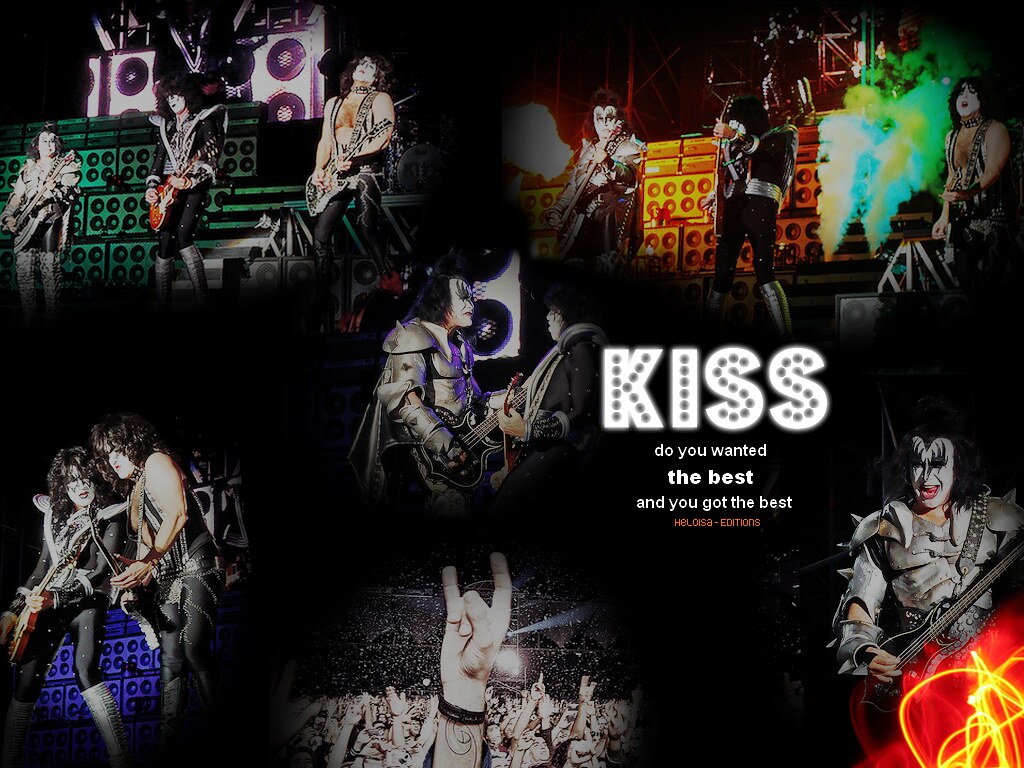This is a detailed poster for a KISS concert, prominently featuring the band's iconic imagery and slogan. At the center right of the black background, "KISS" is boldly displayed in large white block letters, with smaller black-dotted letters inside, reading "KISS." Below this, in bold white text, it states "Do you wanted the best," followed by "and you got the best" in regular white text. Additionally, there's orange text that appears to say "HELLOWESSA EDITIONS."

Surrounding this central text are six circular-framed concert photos, emphasizing the energy and theatrics of a KISS performance. The top right and top left images each show all three band members in full makeup and colorful outfits, playing their guitars under the concert lights. Gene Simmons, identifiable by his signature makeup with white face paint and black spikes around his eyes, appears in the middle photo, sporting a purple necklace, and again in the bottom right image, enhanced by a swirling neon light effect. The bottom center photo captures the audience’s enthusiasm, with a fan displaying the rock and roll hand sign – index and pinky fingers raised – amidst a sea of raised hands. Lastly, the bottom left photo showcases Paul Stanley with another band member, both dressed in their distinctive black leotards and silver boots, engaged in a dynamic stage performance.